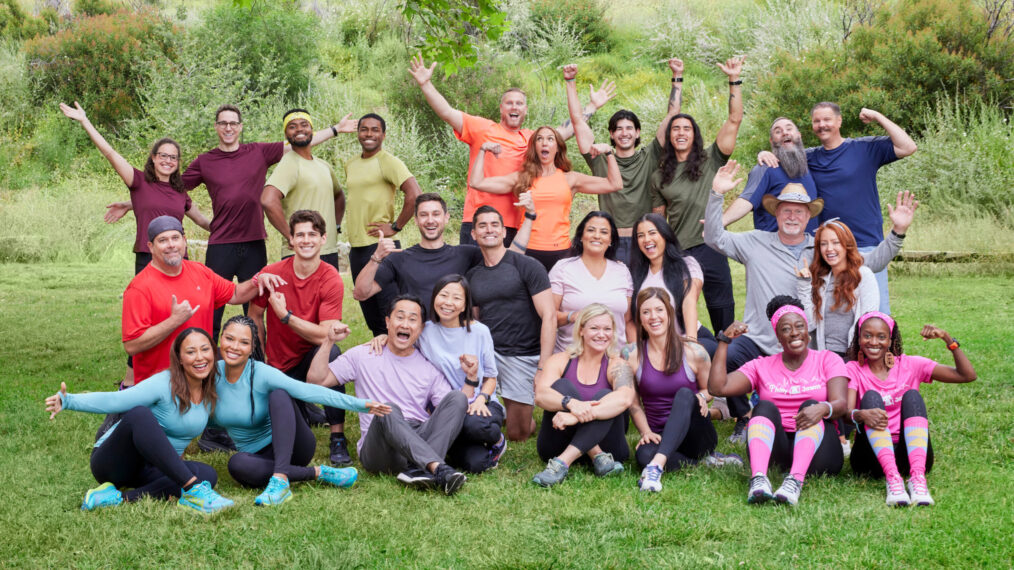This is a vibrant and spirited group photograph featuring 26 people arranged in pairs, each wearing matching athletic clothing in a wide array of colors that creates a rainbow-like effect. The pairs are posing outdoors on green grass, with lush trees and shrubs in the background suggesting an energetic and fresh atmosphere. In the front row, there are two women dressed in pink, followed by two women in purple, a group in lilac, then pairs in teal, gray, white, black, and red. Behind them, the pairs continue with colors like burgundy, yellow, orange, olive, and navy blue. The individuals are showing a variety of expressive poses, such as smiling, waving, flexing their muscles, or playfully putting their arms around each other. The photo suggests the start of an exciting journey or competition, filled with energy and anticipation, as the participants look enthusiastic, ready, and full of life.